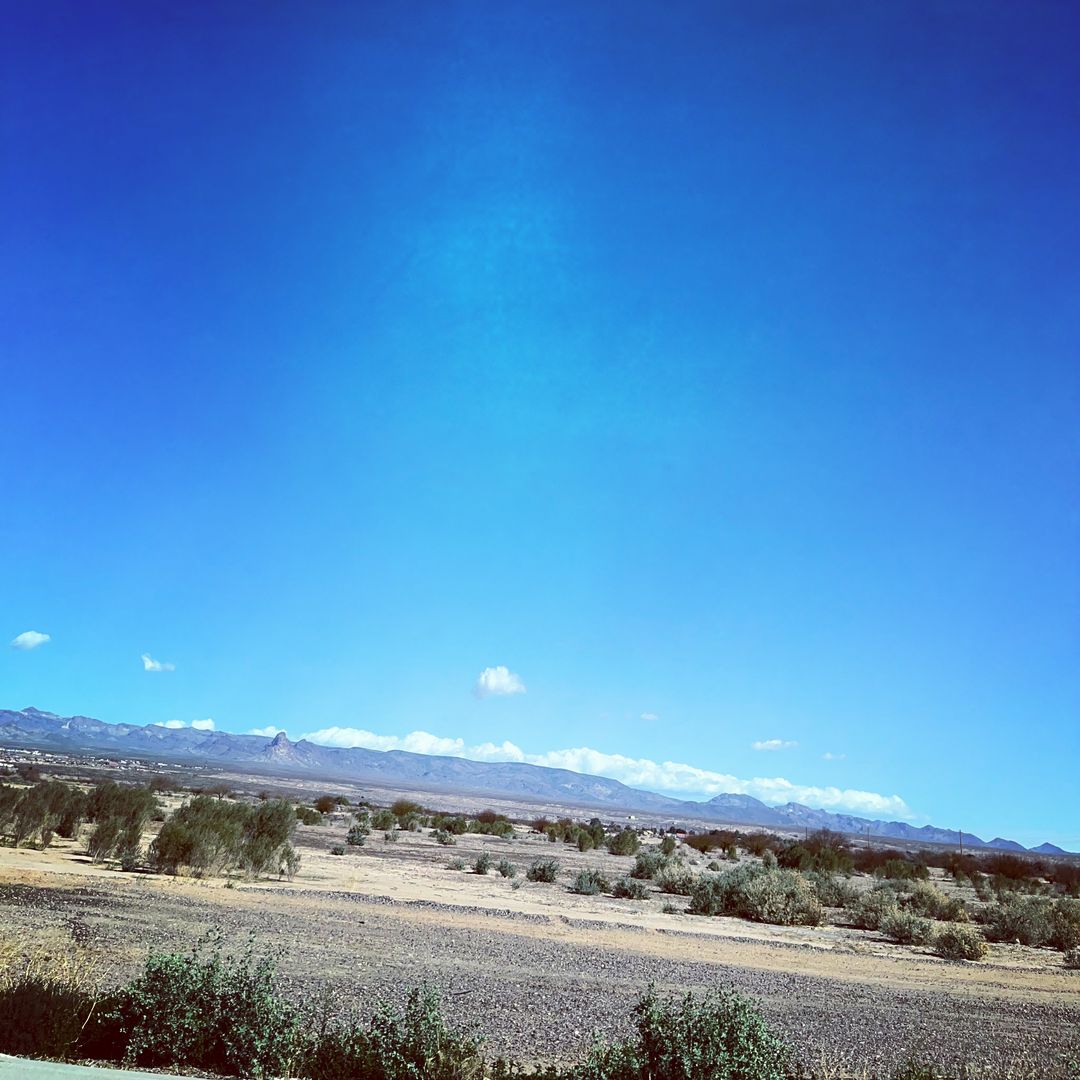This Instagram photo captures a vast desert landscape under a vibrant blue sky that dominates the top 75% of the square-framed image, enhanced by a nostalgic Instagram filter. The backdrop features distant, canyon-like mountains beneath a nearly cloudless sky, interrupted only by a few faint clouds on the horizon. The arid ground below is a mix of beige and tan, appearing dry, hard, and lifeless. Sparse desert plants such as cactuses, muted green shrubs, and small bushes are scattered throughout the scene. A lone road cuts through the barren terrain. Despite minimal, indistinct structures suggested on the periphery, no prominent buildings, animals, or people are visible, emphasizing the vast, empty expanse reminiscent of Death Valley in South California.